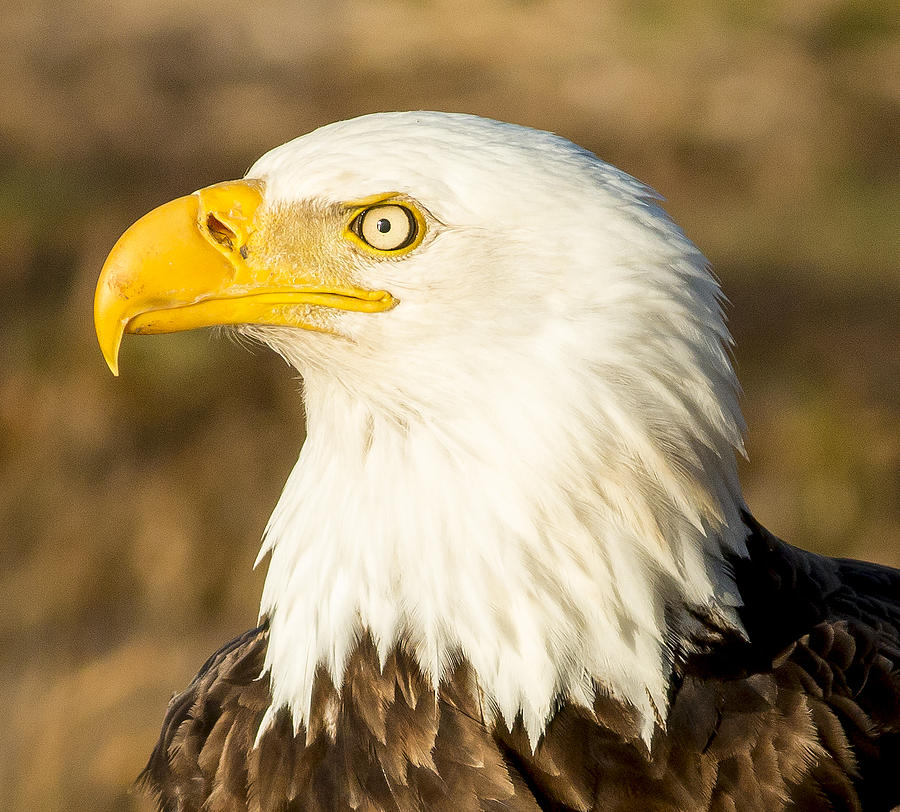This close-up image captures the majestic profile of a bald eagle, its sharply defined features set against a blurred, muddy brown background interspersed with hints of green foliage. The eagle’s head, turned to the left, reveals its striking white feathers and a large, hook-shaped yellow beak shining in the sunlight. The bird's eye, ringed with yellow skin, showcases a white background with a central black pupil, giving it a piercing gaze. The strong lighting accentuates the eagle’s proud, dignified expression. Beneath the head, the neck feathers remain white before transitioning into the darker brown and light brown plumage of the body's shoulder area, which is partially visible due to the image's tight crop. The overall clarity and high definition of the photograph emphasize the eagle's regal appearance and intricate details, from the texture of its feathers to the subtle shine on its beak.